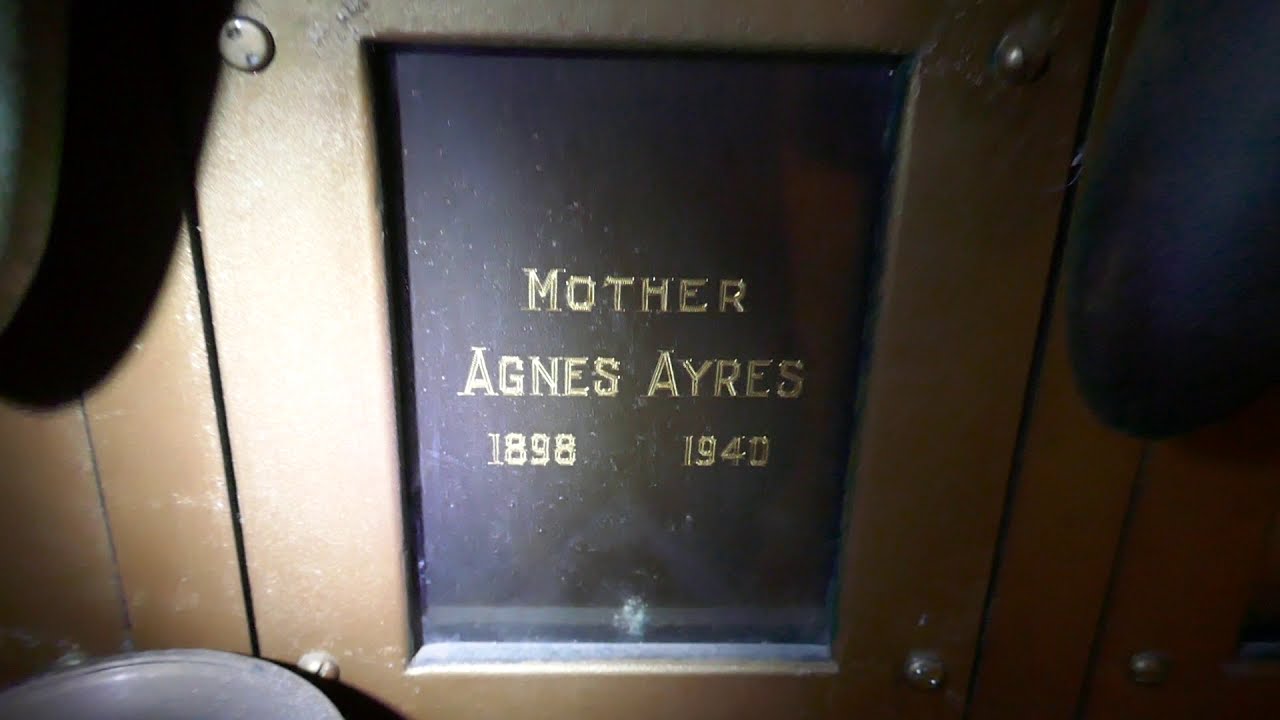The photograph is a color image in landscape orientation, featuring a memorial plaque set into a wooden wall. The central focus of the image is a rectangular, dark brown metal placard with gold-raised lettering. The text is divided into three lines: the first line reads "Mother," the second "Agnes Ayres," and the third line lists the years "1898" on the left and "1940" on the right. This plaque, reminiscent of a gravestone placard, is mounted within a wooden frame, secured by silver hardware at each corner. It appears as part of a row of similar plaques or memorial doors. A light source illuminates the scene from the left, highlighting the detail and texture of the materials.